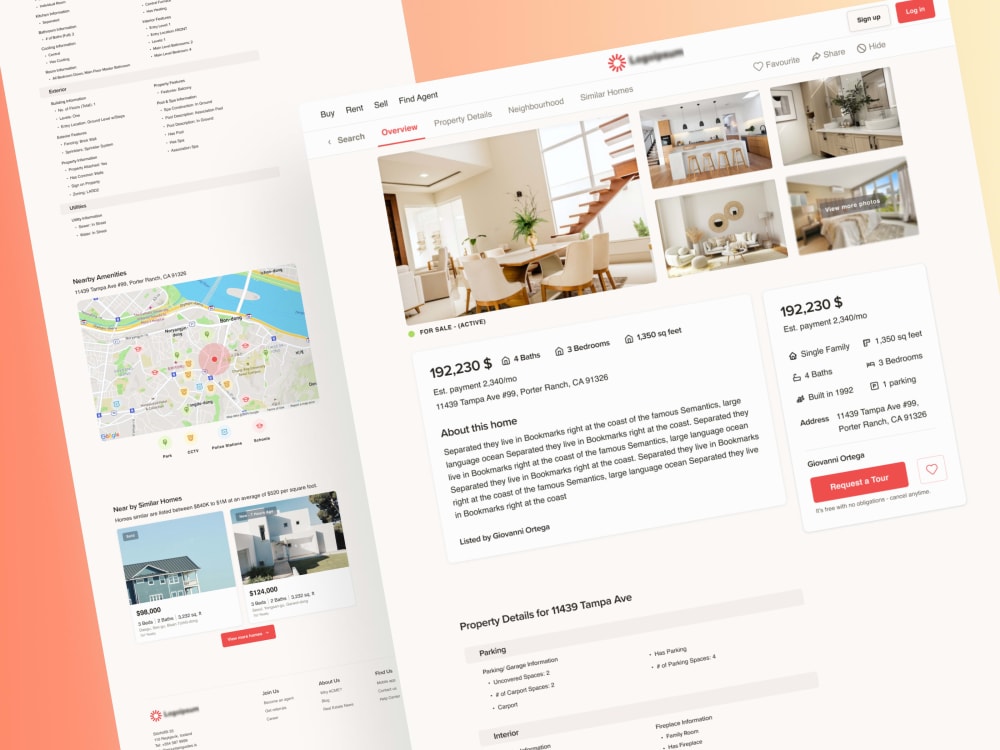This image features a salmon-colored background with a composite of various real estate listing elements. At the top left, there is a small, blurry map with a circled area in pink labeled "Nearby Amenities." Below this, a section titled "Nearby Similar Homes" showcases a photograph of a blue, two-story house. On the right is an image of a white, boxy-style house.

Moving to the right side of the layout, there is a menu bar with options including "Buy," "Rent," "Sell," and "Find Agent." One of the words has been blurred out. The options "Search," "Overview" (which has been selected), "Property Details," "Neighborhood," "Similar Homes," "Favorite," "Share," and "Hide" are visible.

The interior of the house is presented through a series of photographs below this menu. The first image highlights a dining room with a table surrounded by white chairs and a wooden staircase in the background. Additional photos display various rooms: the kitchen, bathroom, living room area, and a bedroom.

Beneath these images, key details of the property are listed:
- Status: For Sale, Active
- Price: $192,230
- Specifications: Four baths, three bedrooms, 1,350 square feet
- Estimated Monthly Payment: $2,340
- Address: 11439 Tampa Avenue, Unit 99, Porter Ranch, California, 91326

A brief, nonsensical placeholder text appears under the "About this Home" section, indicating that this area typically contains a descriptive paragraph about the property.

The listing information at the bottom summarizes the key details and reiterates the address and price, along with the agent's information:
- Listed by: Giovanni Ortega
- Year Built: 1992
- Parking: 1 space
- Request a Tour: It's free with no obligations and can be canceled anytime.